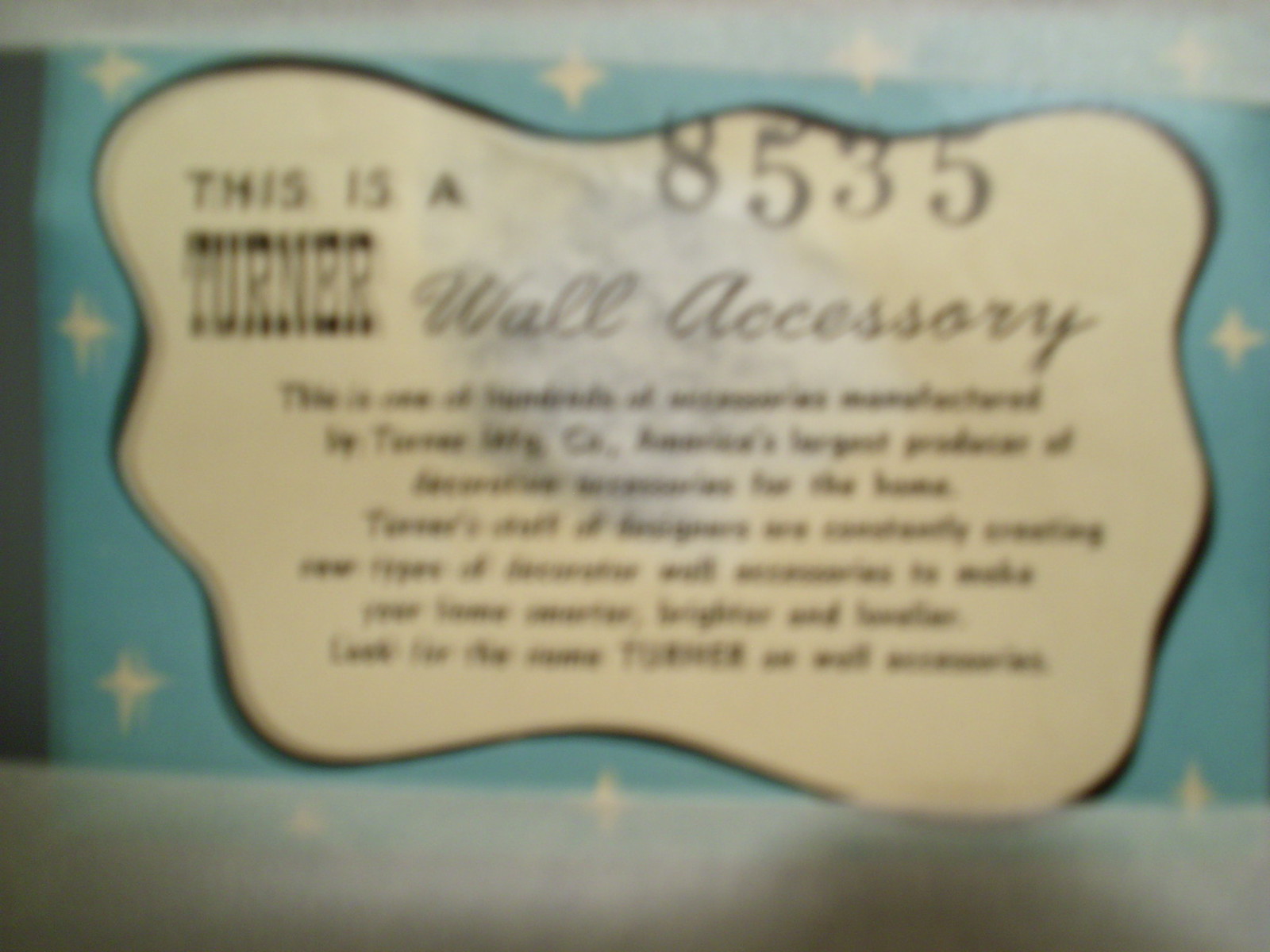This image displays the brightly colored blue and white packaging of a product. The packaging is predominantly a vibrant turquoise blue, adorned with four-pointed white stars scattered throughout. Central to the design is a prominent, wavy-edged, beige label outlined with black, adding a touch of contrast. This wavy label appears more pronounced on the sides and contains a series of black printed text. At the top of this label, there are the numbers 8535, conspicuously positioned as if peeking out. The main text on the label clearly reads, "This is a Turner wall accessory." Below this declaration, a paragraph of text is visible but unfortunately too blurred to be decipherable. The overall presentation suggests a product label designed with eye-catching colors and decorative stars to potentially appeal to shoppers.